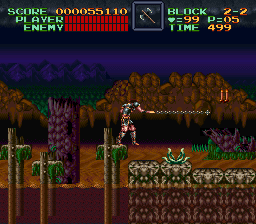This image is a small, square screenshot from a dated video game, likely from the 90s, featuring nostalgic, blocky graphics. At the top of the screen, there are three lines of greenish text: "Score," "Player," and "Enemy," with numerical scores displayed in gold and several red slashes representing player and enemy status. Opposite this, the right side displays "Block: 2-2," "Heart = 99," "P = 05," and "Time = 499" in capitalized letters. The scene captures a male figure, possibly a knight, wielding a weapon or laser device as he moves forward. The figure stands on a tan, barren ground, with a large tree trunk and scattered green plant life. The background shifts to dark brown and darker blue hues, adding contrast, and appears to feature clustered human head-like shapes. The overall aesthetic evokes a setting reminiscent of ancient Persia or Aladdin's world.